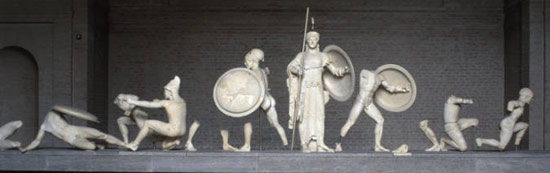The image depicts a black-and-white photo of an assortment of white figurines representing ancient Roman soldiers, displayed on a gray ledge against a gray brick wall. The central figure stands out, brandishing a shield and a long spear or staff, facing forward. Surrounding this figure are others in various states of disrepair and disarray. Some of the statues are headless, one on the far left has dropped its shield to the ground, and there are lone limbs scattered among them. Each figure seems to strike a different pose or action, such as punching or extending a hand, adding to the chaotic scene. The collection appears fragmented, with certain figurines missing significant parts like heads, bodies, or shields, creating an odd and disjointed display of ancient warriors.